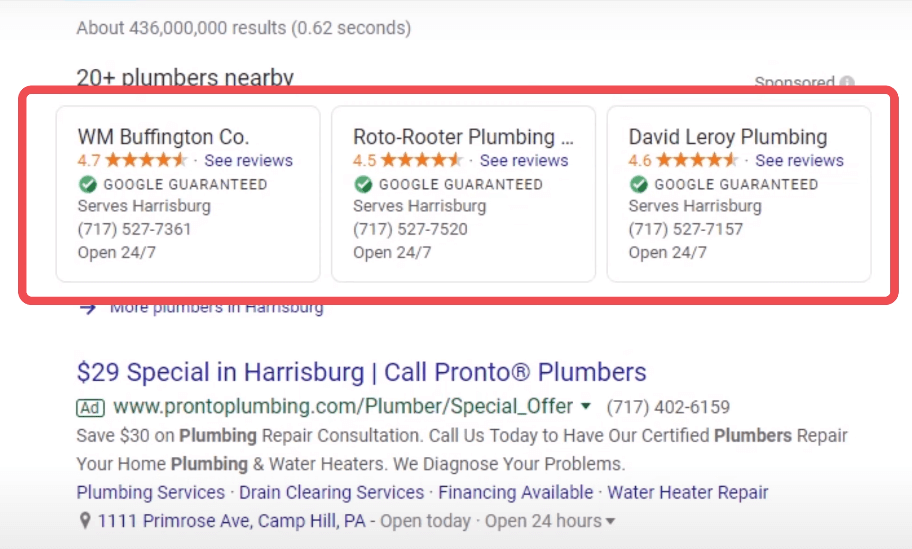The image depicts a Google search results page for plumbers in Harrisburg. At the top, it shows approximately 436 million results found in 0.62 seconds. The first section is a sponsored advertisement featuring over 20 nearby plumbers. Highlighted are three companies: W.M. Buffington Co. with a 4.7-star rating, Roto-Rooter Plumbing with a 4.5-star rating, and David LeRoy Plumbing with a 4.6-star rating. Each listing mentions that they serve Harrisburg and are available 24/7, providing contact numbers for each company. 

Below the sponsored ad, a clickable blue link labeled "More Plumbers in Harrisburg" offers additional options. Following this, another ad appears masquerading as a search result. It promotes Pronto Plumbers in Harrisburg with a $29 special. A green "Ad" box precedes the company's link, followed by a phone number in black text. Further down, more black text elaborates on the company's services. The ad concludes with blue hyperlinked keywords such as "Plumbing Services," "Drain Clearing Services," "Financing Available," "Water Heater Repair," and the company’s address.